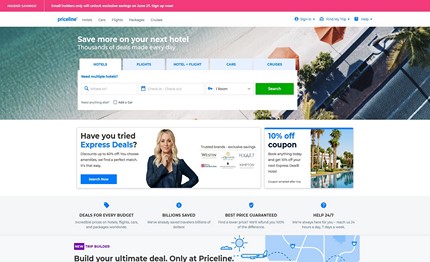**Descriptive Caption:**

The image is a screenshot from a website’s homepage, oriented in landscape and somewhat small, making details hard to discern. At the top of the screenshot, there is a pinkish horizontal rectangular banner with white text. Below this, there is a white horizontal rectangular box without borders, containing text. Within this box, a blue logo prominently displaying "Priceline" is visible, accompanied by several smaller, unreadable black buttons to its right, and three clickable blue objects on the far right.

Directly beneath this section, a long, narrow rectangle spans across the screen, featuring a close-up image of a hotel. Superimposed on this image is a white pop-up box with tabs for searching and customizing options.

Further down, there is another horizontal white rectangular border. Inside this border, on the left, is an image of a blonde woman wearing a black shirt, accompanied by text that says, "Have you tried Express Deals?" The phrase "Express Deals" appears in blue, and next to it is a clickable blue box with white text. To the right of this section, an image showcases a hotel and a pool, along with text offering a "10% off coupon."

At the bottom, a gray box features several clickable blue icons, with black text underneath that reads, "Build your ultimate deal only at Priceline." This text is followed by a blue "Priceline" logo.